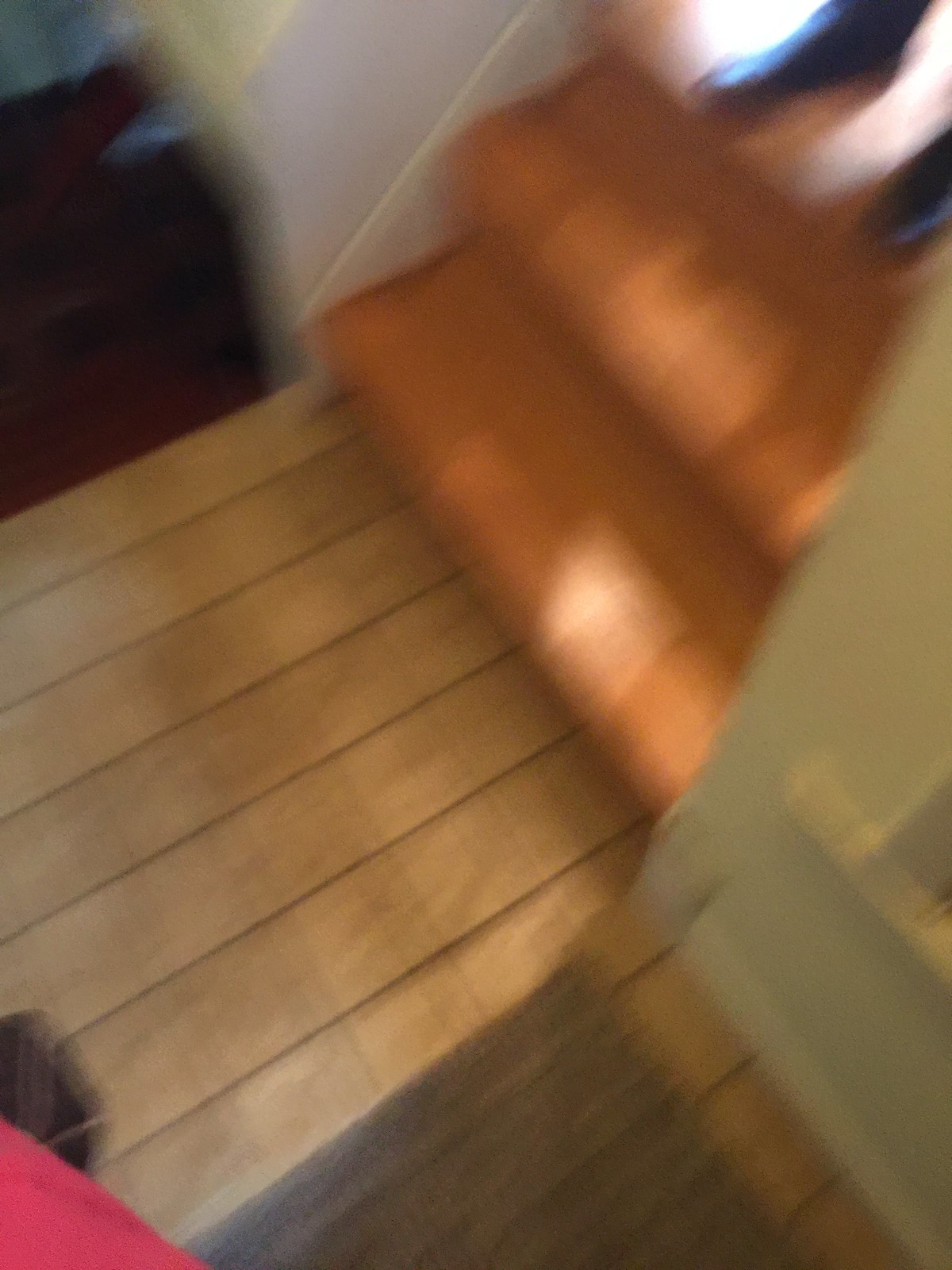A blurry photograph captures the descending perspective of a staircase. The staircase, constructed from brown wood, leads down to a tiled floor of a slightly different brown hue. At the base of the stairs, a rug spreads out on the floor. In the upper right corner, a pair of black shoes rests on the third step, hinting at someone's presence. A piece of red fabric is visible in the bottom left of the frame, adding a splash of color to the image. The overall blurriness of the photograph lends it an abstract, almost mysterious quality.